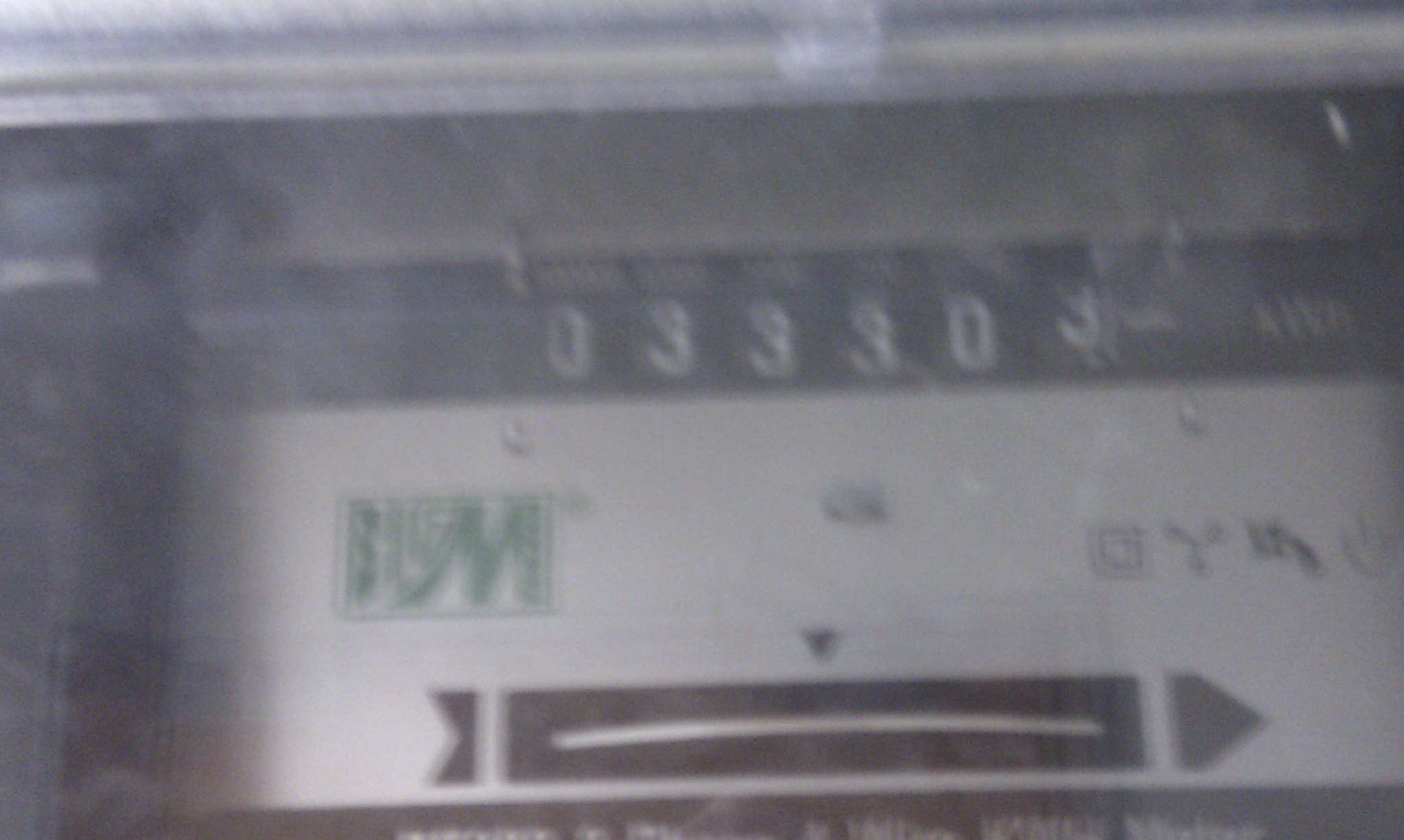This photograph captures a blurred image that likely depicts a numerical interface, possibly from a train station, airport, or even a car's dashboard. The central focus is on the white numbers "033 303" set against a black background. These numbers seem to be part of a meter or odometer, as the last digit appears to be rolling over. The image is hazy, possibly due to a reflective plastic screen or a dirty window obstructing a clear view. An arrow pointing to the right is visible below the numbers. In the left section of the image, a green square contains a backward "M" or similar symbol. There are other indistinct letters and symbols scattered around, adding to the complexity of the scene. The photograph does not include any people, time, date, or specific location details, making it challenging to definitively identify the context or purpose of the display.